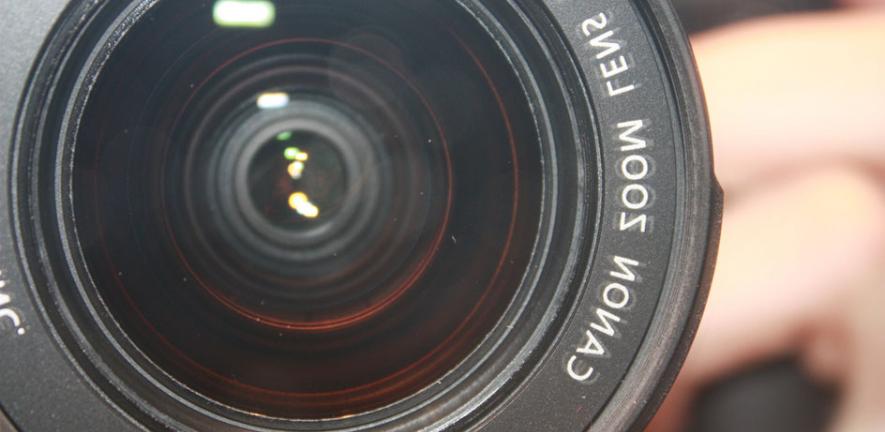This close-up photograph captures the intricate details of a Canon zoom camera lens. The lens dominates the foreground with its dark gray, almost black tone, and circular structure that leads into a series of diminishing concentric circles, giving a tunnel-like appearance. The shiny glass of the lens reflects subtle highlights, featuring glares of green and yellow light, as well as some possible fingerprints. Written in white text on the right side of the lens is "Canon Zoom Lens," although it's presented in reverse due to the angle of the photo. There's also partial, indistinct text on the left side. In the blurred background, a person's fingers can be seen grasping the camera, emphasizing the expensive and professional nature of this piece of equipment. This lens, likely an add-on accessory, showcases its premium build and the careful engineering typical of Canon products.